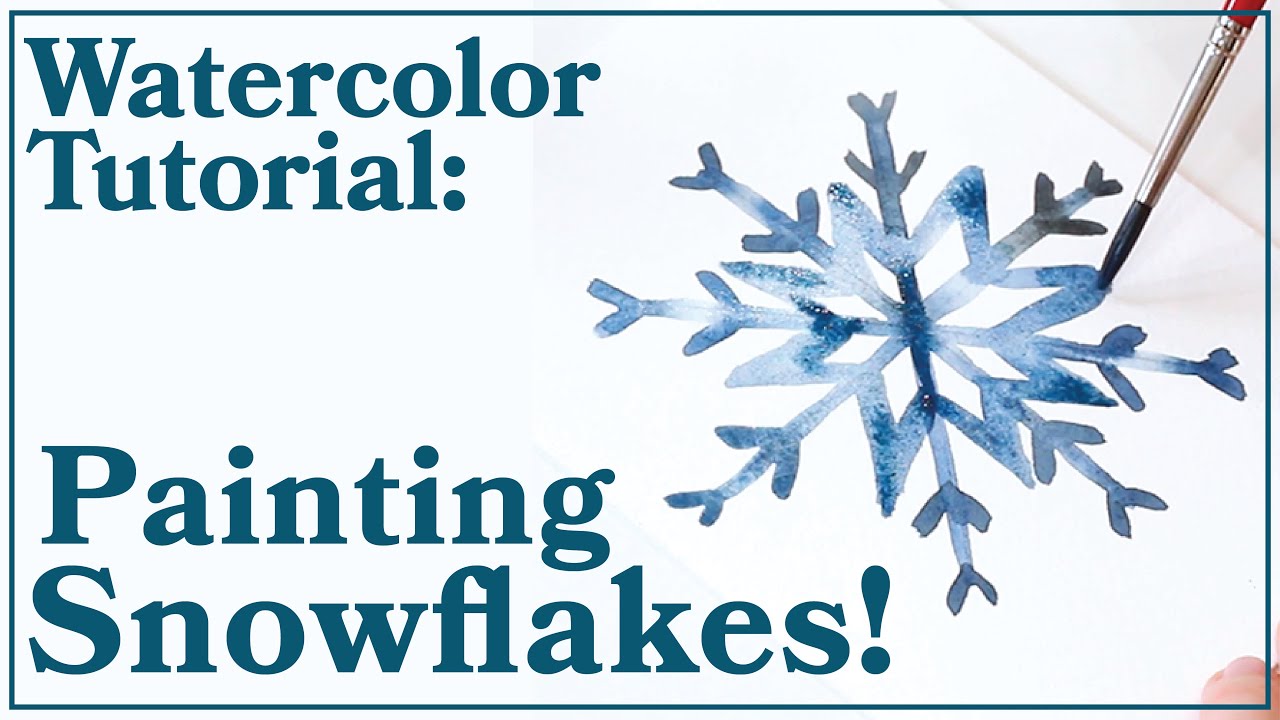This rectangular, horizontally-oriented sign features a thin teal border and prominently announces a Watercolor Tutorial on Painting Snowflakes. On the left side, in large teal Times New Roman font, the words "Watercolor Tutorial" appear at the top, followed by "Painting Snowflakes!" below. To the right, a blue and white snowflake is depicted, being meticulously painted by a red-handled brush with a silver front and a black tip, emerging from the upper right corner. The brush seems to be a photographic element, along with a partial view of a hand, indicating the active process of watercolor painting on white watercolor paper.